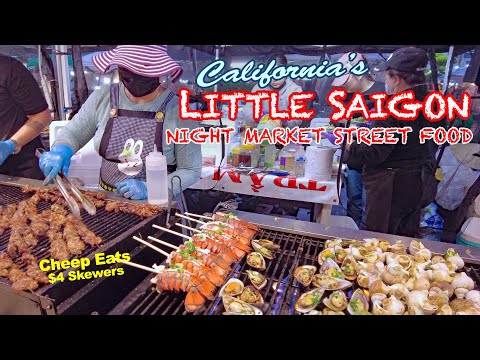The image is an advertisement for California's Little Saigon Night Market Street Food, prominently featuring text in the upper right-hand corner. "California" is elegantly scripted in light blue cursive, while "Little Saigon Night Market Street Food" appears in bold red and white, all caps, non-cursive font. In the lower left corner, bold yellow text reads, "Cheap Eats $4 skewers". The vibrant photograph captures the bustling atmosphere of the market with several cooks working diligently at a grill. The grill is laden with an array of mouth-watering skewers, including chicken, lobster tails, mushrooms, and half-shell oysters. The chefs are seen wearing blue nitrile gloves; the chef on the left is partially visible, wearing a black t-shirt, and the chef next to them is more prominently visible, dressed in a gray long-sleeve shirt, a black apron, a distinctive purple and white striped floppy sun hat, and a black face mask. The energetic scene is further populated with other patrons and cooks bustling in the background, immersing viewers in the lively street food culture of Little Saigon.